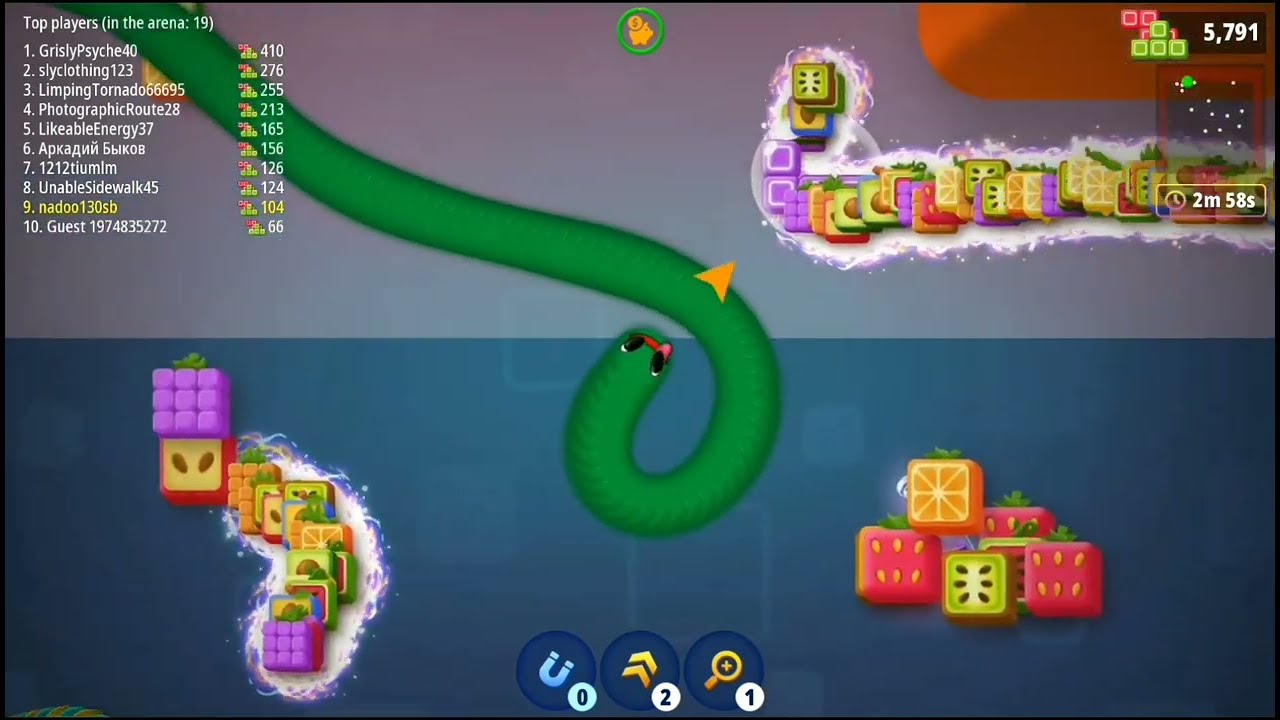The image portrays a colorful screenshot from a mobile game resembling a modern take on Snake. The screen is split into a purple upper section and a blue lower section. Dominating the center is a green snake-like creature with a small face, eyes, and mouth, curling into the scene from the upper left. The snake curves downward and then its head points towards the top right.

In the top-left corner, a leaderboard displays "Top Players in the Arena: 19," listing the top ten scores, with the player "NAD-00130-SB" highlighted in yellow, indicating the current player. Grizzly Psych holds the top position with a score of 40. Opposite, in the top-right corner, colorful Tetris-like blocks form a row, accompanied by a score of 5,791 and a timer showing 2:58.

The game's visual appeal is enhanced by various small fruit-like cubes scattered around the screen, including oranges, strawberries, kiwis, avocados, and grapes. These cubes glow with an energetic aura, especially accentuated in clusters on the bottom right and upper sections. Additional fruit cubes are arranged in a candy cane-like shape across the middle to the right side of the screen. The lower part of the screen also contains an assortment of these vibrant cubes, augmenting the game's engaging and dynamic interface.